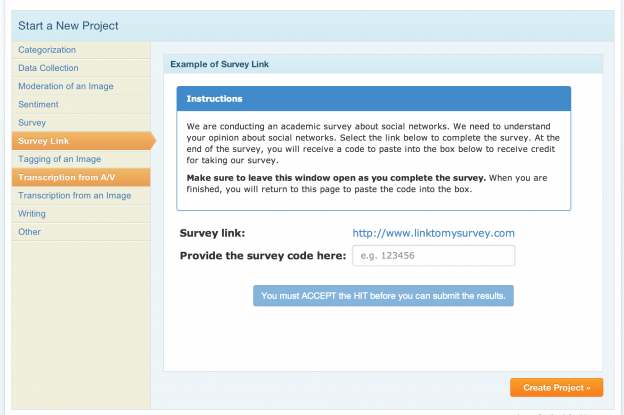The webpage is designed for initiating a new project. At the top left, there's a blue-titled section labeled "Start a New Project." On the left sidebar, there are various tabs, including:

1. Character Categorization
2. Data Collection
3. Image Moderation
4. Sentiment Analysis
5. Survey Link
6. Image Tagging
7. Transcription from Audio/Video
8. Transcription from Image
9. Writing
10. Others

Currently, both the "Survey Link" and "Transcription from Audio/Video" tabs are highlighted in orange, creating some ambiguity about which tab is active.

The main content of the page pertains to creating a survey link. Titled "Example of Survey Link," it includes a blue information box with the following instructions: 
"We're conducting an academic survey about social networks. We need to understand your opinion about social networks. Select the link below to complete the survey."

Below these instructions, there is a field labeled "Survey Link," which contains a URL: [www.linktosmysurvey.com](http://www.linktosmysurvey.com). There is also a text box for entering a "Survey Code," followed by a blue button with a prompt: "You must accept the HIT before you can submit the results." At the bottom right of the page, there's an orange button labeled "Create Project."